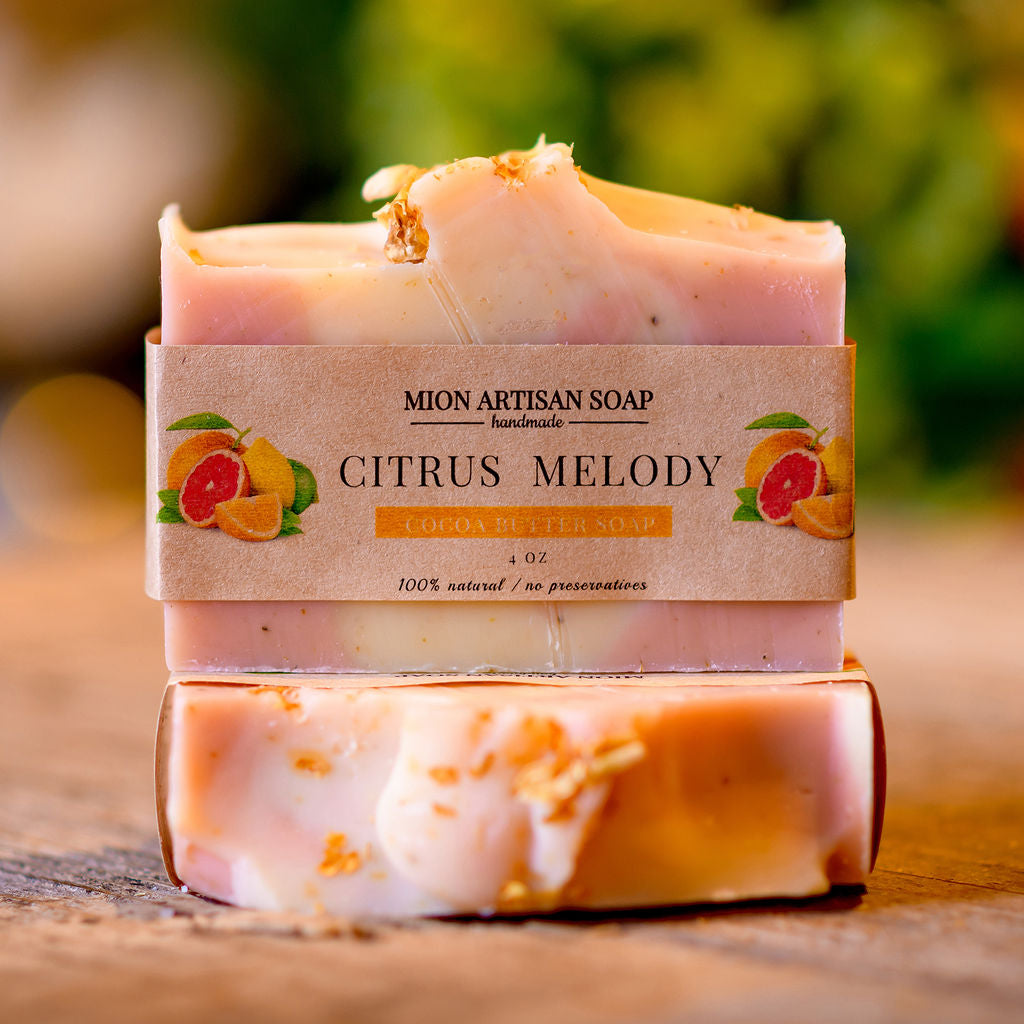This detailed image showcases a bar of Mion Artisan Soap, an exquisite handmade soap with a Citrus Melody scent. The soap, which exudes an enticing blend of orange, yellow, and pink hues, sits atop a wooden surface, further complemented by an out-of-focus green background. The soap is wrapped in an orange-yellow cardboard sleeve featuring bold white lettering. The label prominently displays "Mion Artisan Soap, Handmade" followed by "Cocoa Butter Soap" across the yellow-bordered section. The packaging also provides essential details: "4 oz," "100% natural," and "No preservatives." The wrap is adorned with vibrant illustrations of lemons and grapefruits—lemons are depicted whole and in yellow, while the grapefruits have an orange exterior and a red-pink interior. The soap bar itself, with its peach and cream colored swirls, sits atop another horizontally placed bar of the same luxurious soap.